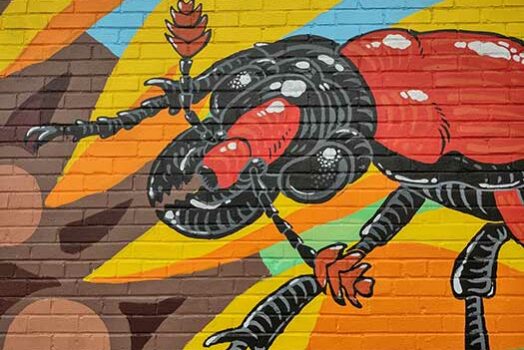The image showcases a vibrant mural painted on a brick wall. The central figure of the mural is a large, menacing bug, possibly a beetle or an ant, with a strikingly vivid red body and a black head adorned with prominent black antennae that end in red, pine cone-shaped feelers near its "nose" area. This creature is depicted in an aggressive stance, appearing poised to attack or move forward. The mural features a rich, multicolored background filled with shades of yellow, orange, blue, green, and brown. Among these colors are what seem to be flower petals and a central circular brown object, suggesting the giant bug may be heading towards these flowers, potentially in search of food. The intricate details and bold colors make the mural a captivating piece of street art.